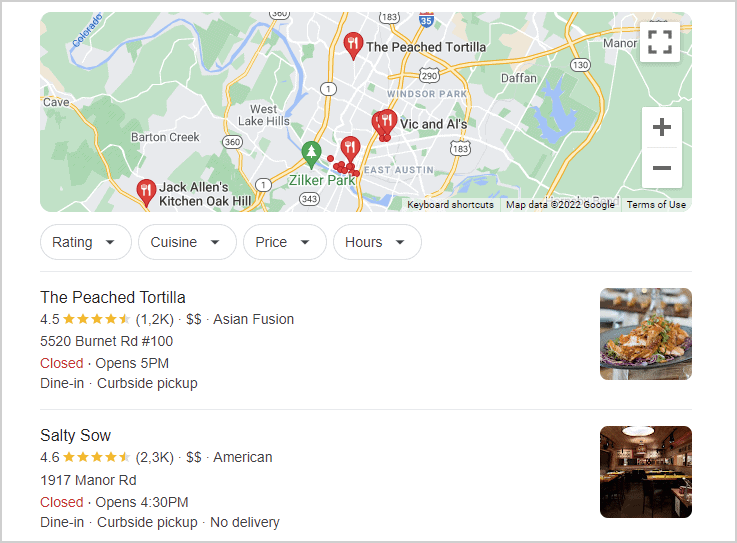A screenshot of Google Maps displays an urban area with multiple eating establishments marked by red arrows featuring a fork and knife icon. Highlighted restaurants include The Peach Tortilla, Vic and Al's, and Jack Allen's Kitchen, Oak Hill, with regions designated as Defan, East Austin, Westlake Hills, and Barton Creek. Major roadways indicated are 183, 290, and Interstate 35.

Below the map, there are four selectable buttons with drop-down options for rating, cuisine, price, and hours. Two restaurant listings are prominently visible. 

First, The Peach Tortilla, which shows an image of a plated dish on the left. It has a four and a half star rating, falls under the $$ price category, and details that it offers dine-in and curbside pickup services. It is currently closed but will reopen at 5 PM.

Second, Salty Sow, with an image displaying the restaurant's interior beside the listing. It has a rating, the number of reviewers, price estimate, and type of cuisine listed. It is also closed but will reopen at 4:30 PM. The services it offers include dine-in and curbside pickup, but no delivery.